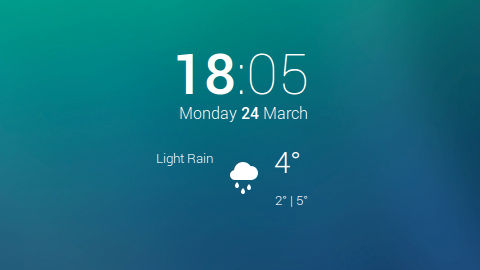The image showcases a digital display that features the current time, date, and weather conditions with a sleek, modern design. The background is a gradient of bluish-green transitioning to teal, reminiscent of the clear, serene waters of the Caribbean. Prominently displayed in white, the time reads "1805," with the "18" in bold for emphasis. Directly below, the date is presented as "Monday, 24 March," with the "24" also bolded for clarity. The weather condition is described as "light rain," accompanied by a minimalistic icon of a white rain cloud with three droplets illustrating rainfall. To the right of this icon, the current temperature is indicated as "4°C," also in white. Beneath this, the forecasted low and high temperatures are displayed as "2°C / 5°C." The overall layout, color scheme, and information suggest that this is likely a weather and time widget designed for a digital device such as a smartphone or computer, providing users with a convenient and visually appealing way to stay informed about their environment.